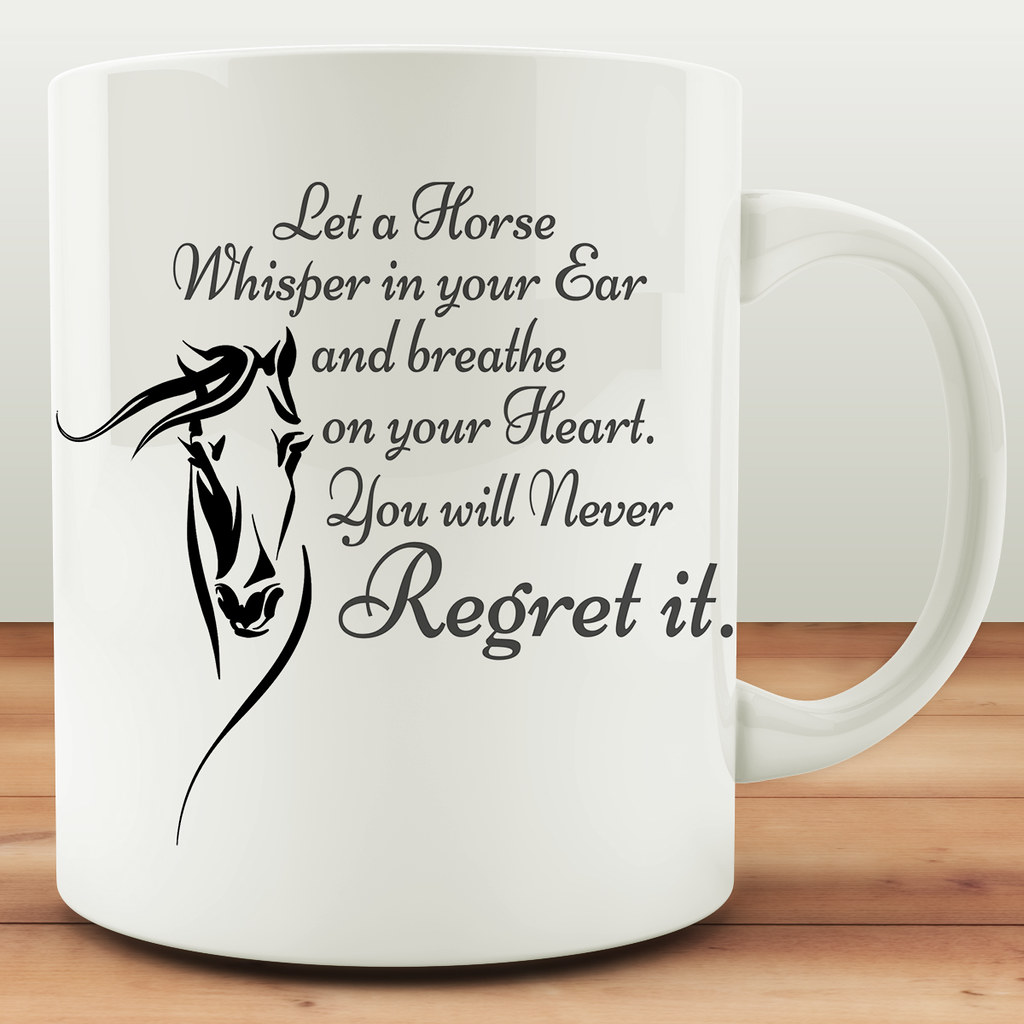This close-up photograph showcases a shiny, white mug on a brown wooden surface against an off-white wall. The handle of the mug is positioned to the right, extending out at a precise 90-degree angle, and features a thin line running through its center. The focal point of the image is the black and light gray text on the mug, which reads, “Let a horse whisper in your ear and breathe on your heart. You will never regret it.” To the left of the text is an artistic, black graphic of a horse's face, with its mane flowing elegantly to the left. The horse's nose is depicted with artistic lines, one extending below its mouth and the other curving and flowing down. The words "regret it" are emphasized in a slightly larger font, underlining the importance of the message. The photograph does not include any liquid or a person holding the mug, emphasizing the design and inspirational saying.